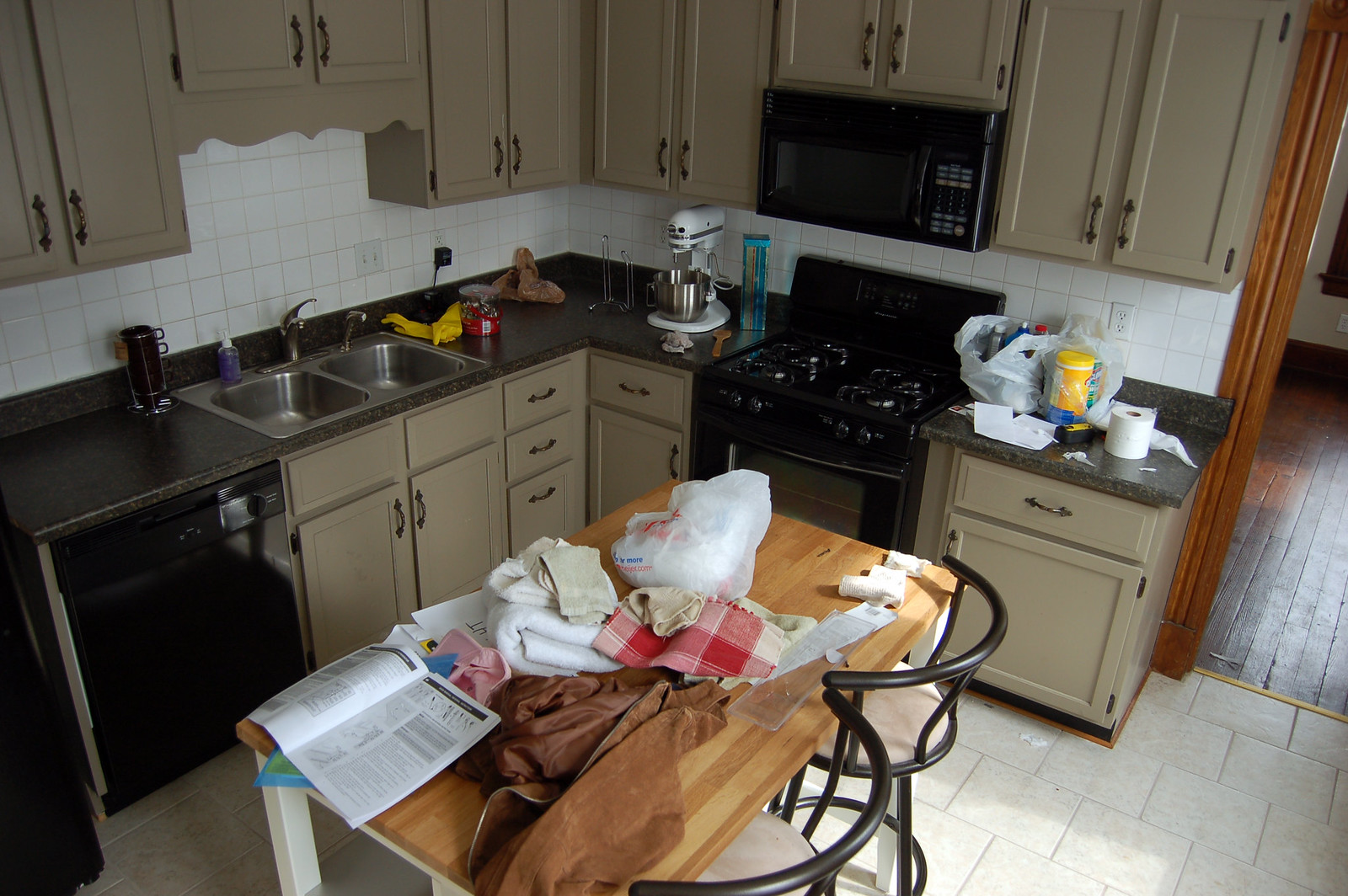This is an image of a cozy kitchen in what appears to be a city apartment with an older style. The kitchen floor is covered with linoleum, while the adjacent room, visible through a doorway framed with wood, has a wooden floor. The kitchen features dark beige cabinets adorned with wrought iron handles, which contribute to the vintage aesthetic. 

The countertops are either quartz or marble, characterized by a dark brown color with striking gold flecks. A black gas stove with an oven is centrally located, and directly above it is a microwave, with more of the dark beige cabinets encircling this area. 

Between the sink and the stove, there is an "elbow" section of the countertop, maximizing the use of space in this compact kitchen. Storage cabinets are positioned below all the countertop areas. On the countertop adjacent to the stove, there is a grocery bag filled with cleaning supplies, including Clorox wipes, toilet paper, and several other miscellaneous items like tools and loose papers, lending a somewhat cluttered appearance. 

On the other side of the stove, a stand mixer sits next to an open box of spaghetti, a wooden spoon, and a rag. A paper towel holder is also present, unfortunately empty. Overall, the kitchen showcases a blend of functionality and a touch of disarray, reflecting the everyday liveliness of urban apartment living.